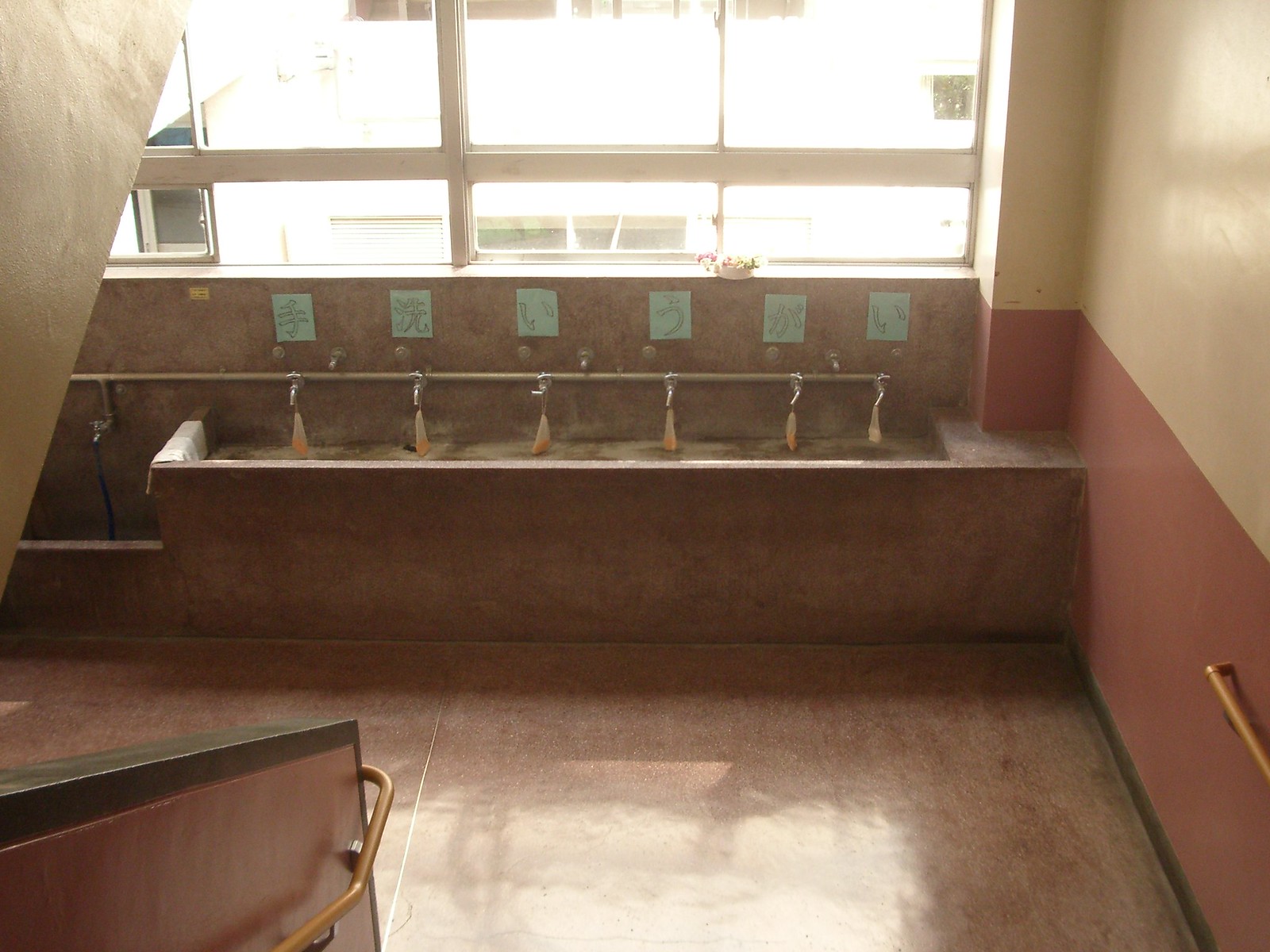The photograph depicts the interior of a public school in Japan, specifically within a stairwell area. The bottom half of the stairwell walls are painted a terracotta color, while the top half is peach. On the right, a handrail made of light-colored wood is visible. The floor at the bottom of the stairs is tan, matching the reddish-brown banister and floor of the stairwell. 

In front of the stairwell, there is a long, dark brown counter that appears to be a communal sink area lined with silver-colored faucets. The water coming from the faucets is discolored, appearing reddish-brown, suggesting neglect or abandonment. The wall above the faucets is adorned with green tiles featuring kanji characters, and there are signs with various drawings. A white-framed window at the end of the stairwell offers a view of a white building outside.

This setup reflects the customary practice in some Japanese public schools where students participate in cleaning and serving each other, though the poor condition of the faucets indicates a lack of recent use or maintenance.